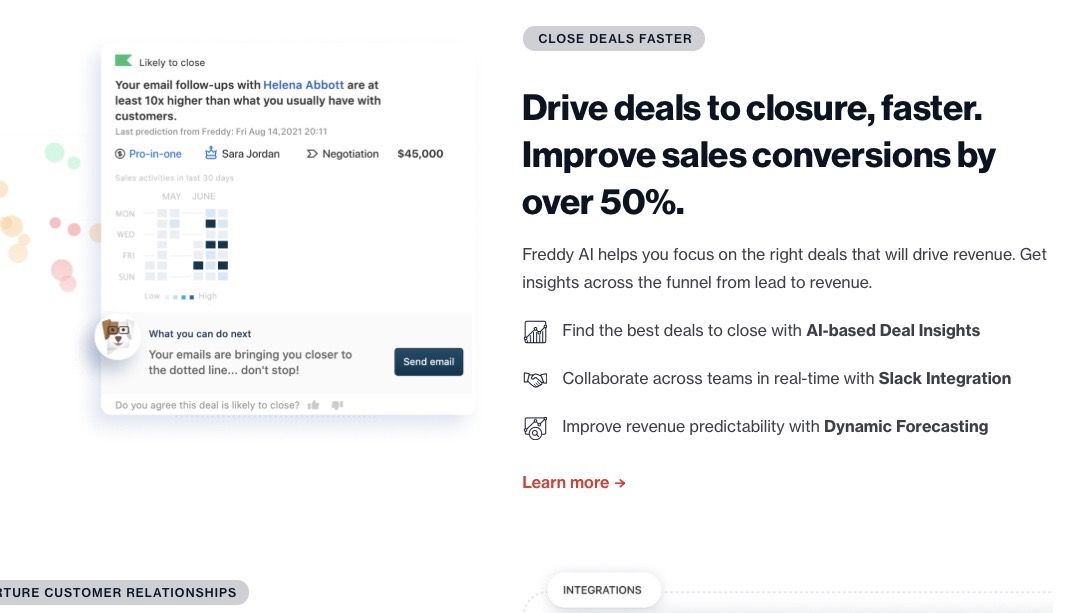**Detailed Caption: Effective Customer Interaction Tool Advertisement**

The advertisement centers on a tool designed to enhance customer interactions and streamline sales processes. On the left-hand side, a visual array of circles in varying hues of green, orange, pink, and yellow catches the eye, reminiscent of a color-coded activity chart.

An outlined box marked "Likely to Close" prominently displays a green flag with trimmed edges. In this box, it states: "Your email follow-ups with Helena Abbott," highlighting Helena Abbott's name in vibrant blue. It emphasizes that the follow-up rate is at least ten times higher than the usual customer interactions.

A timestamp below reads, "Last prediction from Freddie, Friday, August 14th, 2021, at 8:11 PM (or 20:11)." An actionable link labeled "Pro in one" appears in this section. The name Sarah Jordan, accompanied by what looks like a crowned icon (which could also be a birthday cake), adds a touch of personalization.

A rightward pointing arrow labeled "Negotiation" reveals a deal amount of $45,000. Adjacent, a grid tracking "Sales Activities in the Last 30 Days" contrasts May and June against the days of the week: Monday, Wednesday, Friday, and Sunday. Colored boxes focus selectively on a few specific days: one box on Tuesday, two on Thursday, and two on Saturday.

Under a section called "What You Can Do Next," a charming cartoon-like dog is featured. The dog is predominantly white with a brown ear and a patch around its left eye. A motivational message reads: "Your emails are bringing you closer to the dotted line... don’t stop," accompanied by a dark blue "Send Email" button with white text.

The bottom dialogue prompts, "Do you agree that this deal is likely to close?" with some indistinct characters nearby.

On the right-hand side, a gray oval headline, "Close Deals Faster," captures attention. It details benefits such as enhancing sales conversations by over 50% and highlights Freddie AI’s capabilities in focusing on the most promising deals to maximize revenue. Insights are offered from lead inception to final revenue.

Supporting images include a handshake for real-time team collaboration via Slack integration and a magnifying glass over a graph illustrating dynamic forecasting improvements in revenue predictability. A red "Learn More" link encourages further exploration.

At the base, a clear "Integrations" button in black text and uppercase letters invites further engagement, emphasizing highlighted features like AI-based deal insights, Slack integration, and dynamic forecasting in bold text.